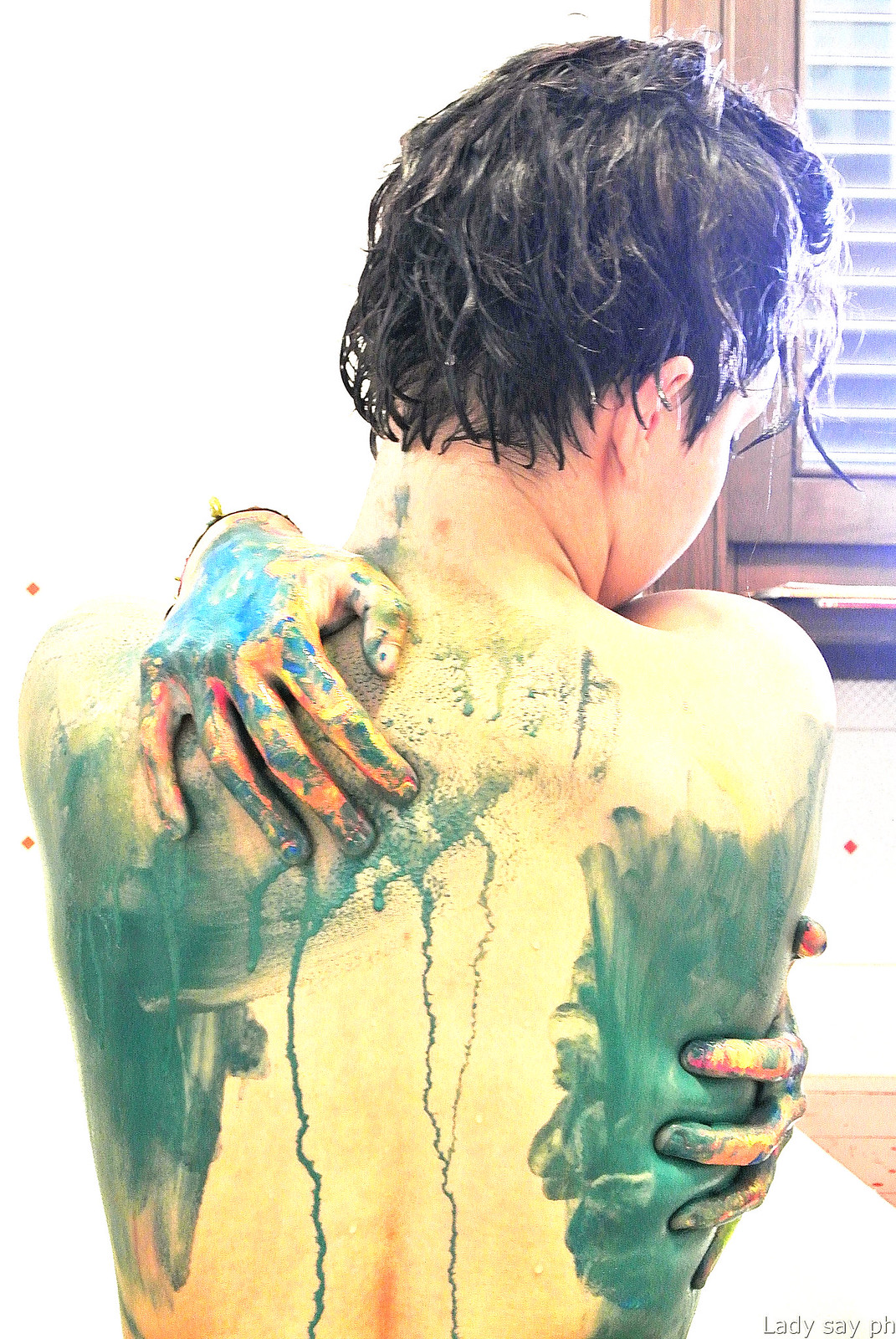The image features a person with short, wet brown hair, facing away from the viewer. The individual's gender is not clearly identifiable, though they exhibit a somewhat feminine appearance. Their arms are wrapped around themselves in a self-embrace: their right arm drapes over their left shoulder while their left hand rests on their right side. The person's back is partially visible, covered in streaks and patches of green, blue, and gray paint that drizzles from the shoulders down to the lower back, adding a surreal texture. Both of the individual's hands are visibly covered in paint, with dark shadows around them enhancing the effect. The upper left quadrant of the image is a stark white, while the background reveals a brown-framed window with white blinds, letting in natural light. At the bottom right corner of the image, there is a caption or text, "Lady say pH," partially overlapping the scene.